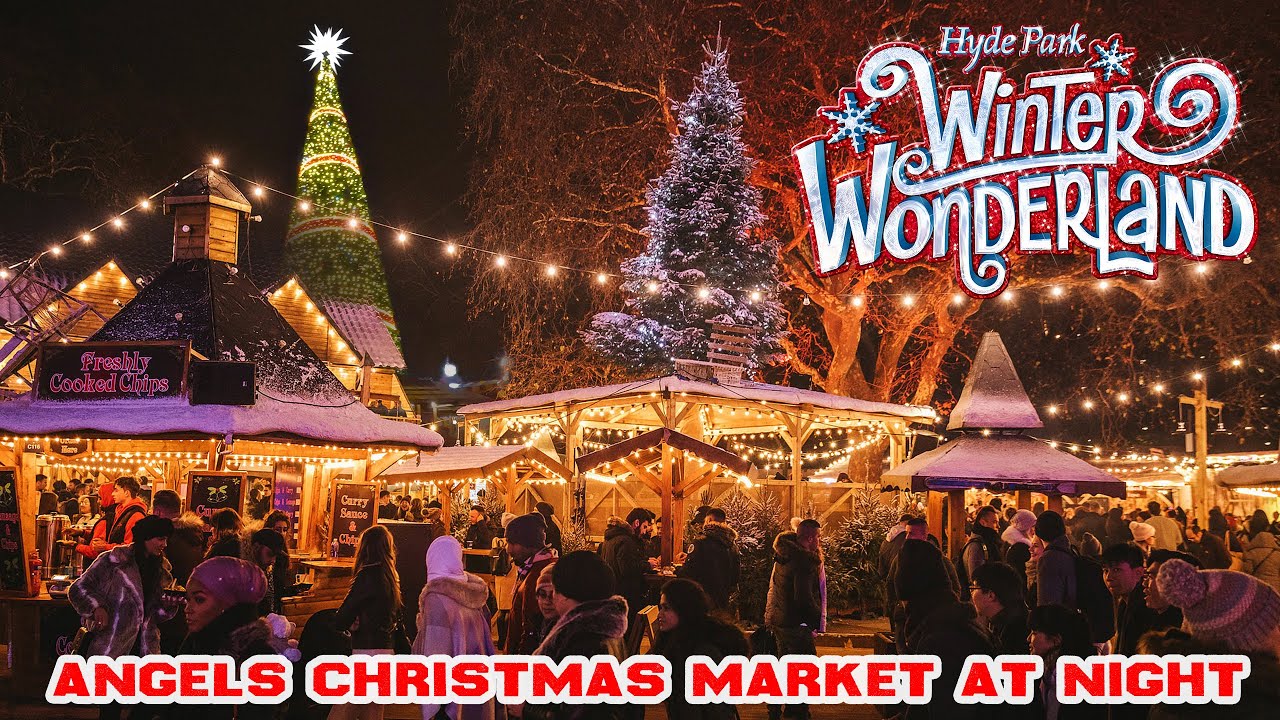This vibrant nighttime image captures the festive atmosphere of an outdoor Christmas market, filled with people dressed in winter wear, all bustling around wooden stalls draped in thick strings of twinkling white lights. The market, identified as Hyde Park's Winter Wonderland, is decorated with an array of Christmas decorations, including several Christmas trees adorned with snow and glistening ornaments. Two standout trees punctuate the scene: one tall green tree on the left, wrapped in red and gold bands with a white star atop, and another silver-lit tree on the right. There are also snow-topped stalls in the middle of the image, contributing to the cozy, warm glow of the setting. The event is further advertised with festive, whimsical lettering that reads "Hyde Park, Winter Wonderland" in a stylized, snowflake-adorned font in the upper right corner, while red text with a white outline at the bottom proclaims "Angels Christmas Market at Night." Overall, the photo exudes holiday cheer and a welcoming winter ambiance.